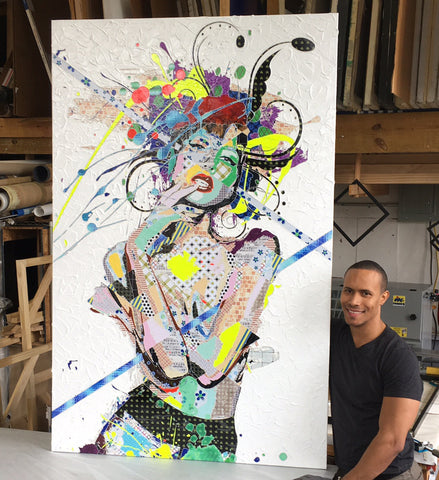In this indoor photograph, we are presented with a striking scene centered around a large, white canvas adorned with a highly stylized and colorful painting of a woman. The painting is modern in style, featuring the woman's hair formed by various splotches of vibrant colors such as red, blue, yellow, and orange. Her face is expressive, with fingers resting contemplatively on her lips and a visible set of teeth beneath dark red lipstick. The abstract nature of the painting continues down her body, blending into multi-colored designs, including a notable black checker pattern.

To the right side of the canvas stands a young African-American man with short, dark hair, dressed in a black t-shirt and gray pants. He is smiling and looking directly into the camera, suggesting pride and joy, likely indicating he is the artist. His arm is positioned beneath the painting, perhaps holding it up. The man is significantly smaller in stature compared to the towering canvas, emphasizing the artwork's grand scale. The background reveals an artist's studio environment, filled with wooden frames, additional canvases perched on a high shelf, and various machinery and materials including what seems to be a wooden easel on the left side behind the painting.